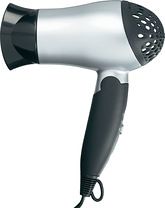This photograph showcases a nondescript, modern-looking hairdryer on a completely white background, reminiscent of product images commonly found on e-commerce websites. The hairdryer is positioned upright with its handle at the bottom, and it is angled to the left. The handle is thin and black, and a cord is visible emerging from its lower end. 

The main body of the hairdryer is silver, while the cap over the air intake, located on the right, is a black plastic casing with holes. The nozzle on the left, where the air comes out, is also black. Additionally, a diffuser is attached to the end of the hairdryer. Control switches are positioned on the back of the handle. The image lacks any brand markings, making it impossible to determine the model or make. Overall, the minimalist and clean presentation emphasizes the hairdryer’s basic design and color scheme, suitable for general use.